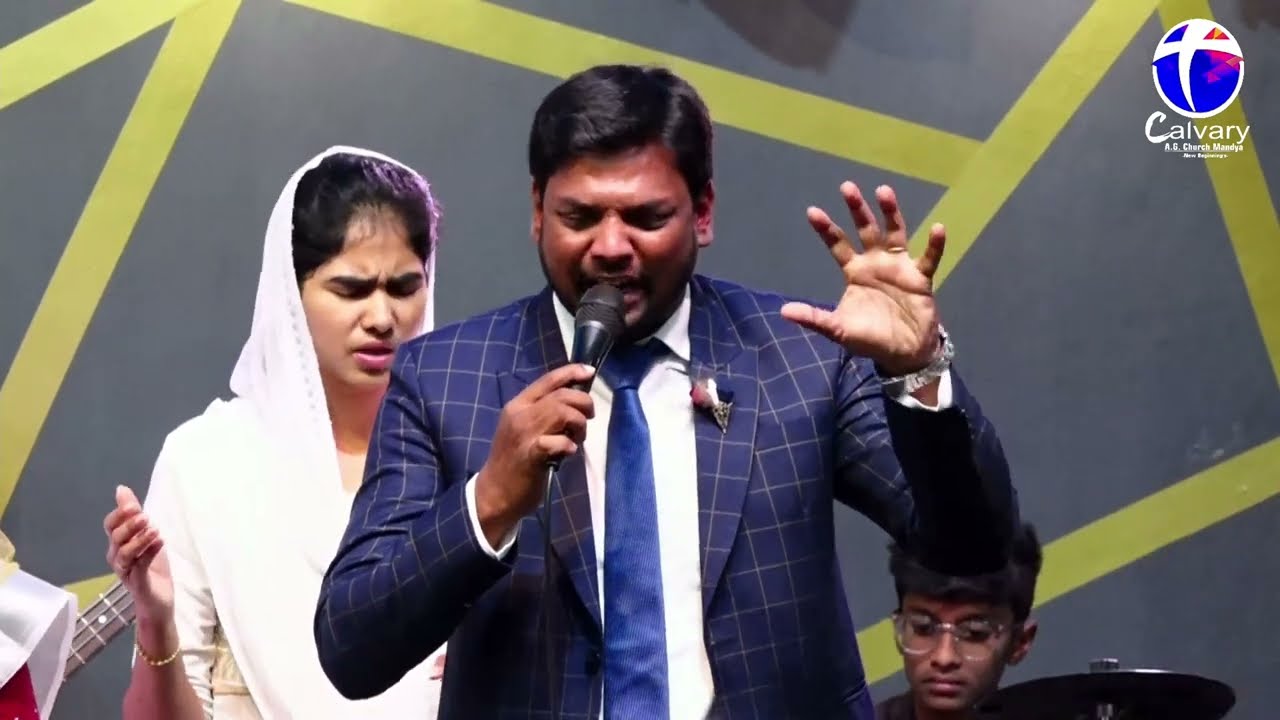In a vivid indoor setting, this photograph captures a lively scene at what appears to be a church event. The focal point of the image is a man singing passionately into a black microphone. He is dressed in a striking blue suit jacket patterned with white lines forming squares, a crisp white shirt, and a navy blue tie. A flower adorns his lapel, adding a touch of elegance. The man, who appears to be of Indian descent with dark hair, is delivering his performance with animated hand gestures.

Behind him, slightly to the left, stands a woman draped in white clothing with a shawl covering her head. Her eyes are closed and her hands are raised in a gesture that suggests prayer or agreement, contributing to the solemnity of the moment. To the right side of the man, a young boy can be seen sitting at a drum set, identifiable by his glasses and the presence of a cymbal.

The background features a gray wall adorned with a pattern of yellow lines. In the upper right corner, a circular logo with a white cross inside stands out, beneath which the words "Calvary AG Church Mandya" are inscribed, indicating the probable location of this heartfelt scene. Overall, the image is rich with spiritual and communal energy, highlighting a moment of deep connection and musical expression.